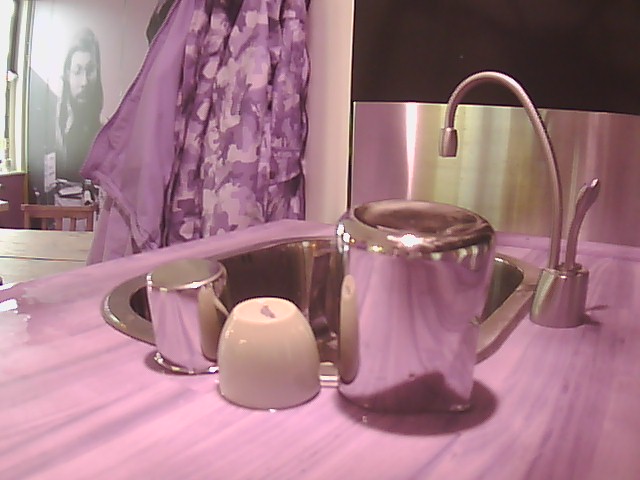This image depicts a room that is difficult to distinguish between a kitchen or a bathroom due to the mixed elements present. The focal point is a shiny, silver sink, possibly a bathroom sink, given the surrounding elements. Adjacent to the sink are three containers: one white cup and two silver cups. The countertop has a unique, wooden texture that appears purple, potentially influenced by the lighting in the room. The surface of the counter seems to be slightly wet.

Hanging on the wall are what look like purple bathrobes, outfits, or jackets, adding to the ambiguity of the room's purpose. To the left of the sink, a black and white picture frame is visible, displaying an image of a woman with glasses. In the background, further complicating the identification of the room, a brown chair and a white table are partially visible. Despite the varying clues, the exact nature of whether this is a kitchen or bathroom remains unclear.